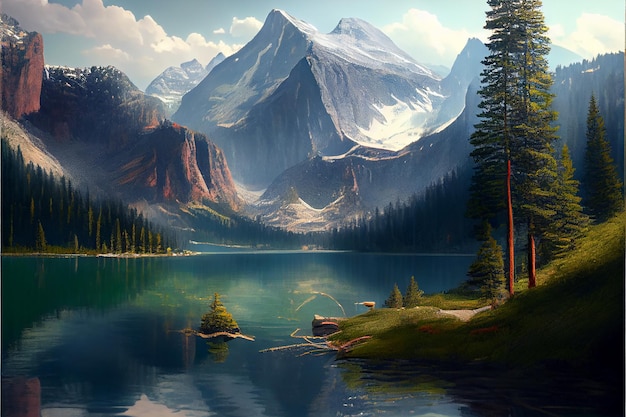The image is a hyper-realistic digital painting reminiscent of a Bob Ross creation. The foreground features a serene, still lake with a blue-green hue. Flanking the lake on the right side is a patch of land with lush green grass and tall pine trees, while the left side also showcases dense evergreen trees. The middle of the image transitions from the rich vegetation to a majestic mountain range in the background. These mountains vary in color, with some sporting a pinkish-brown hue, others rich purple, and a central peak adorned with snow. Topping the highest peaks are dark gray rocks with more snow, emphasizing the elevation. A blue sky filled with fluffy white clouds stretches across the upper part of the image, adding to the peaceful ambiance. The lake’s glassy surface perfectly mirrors the towering mountains and greenery, enhancing the immersive natural beauty of this tranquil scene. There are no visible people or animals, and no text, highlighting the untouched essence of nature captured in this professional-quality artwork.